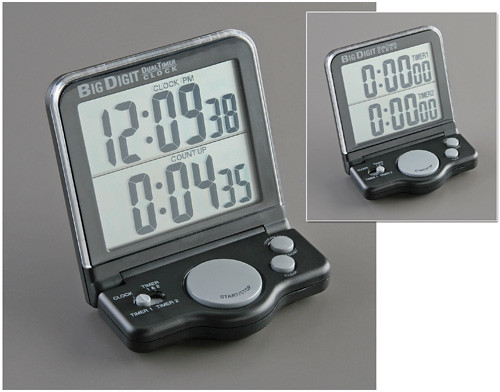This image showcases a compact, portable digital travel alarm clock with a sleek design. The clock features a large square screen and a rounded, minimalistic base that allows it to fold neatly for travel. A prominent characteristic is the folding mechanism where the top part, with a silver border and a gray inner frame, hinges onto the bottom. 

On the main display, above a separating black line, the time reads "12:09:38 PM" and below it, the count-up timer displays "0:04:35". The screen is divided into two sections, labeled "Clock PM" at the top and "Count Up" beneath the line. Notably, the base includes essential controls: on the right side, a slider toggles between 'Clock' and 'Timer' settings, marked with white lettering, while the center has a large, prominent start/stop button. Adjacent to this button are two additional angled buttons, although their labels are not readable.

Overlaying the top right of this primary image is a smaller inset of the same clock, mirroring the larger version but with its display set to all zeros. The background of both images is gray, adding to the modern, streamlined appearance. Lastly, the description on the clock itself, visible in the gray border of the main image, reads "Big Digit Dual Timer Clock".